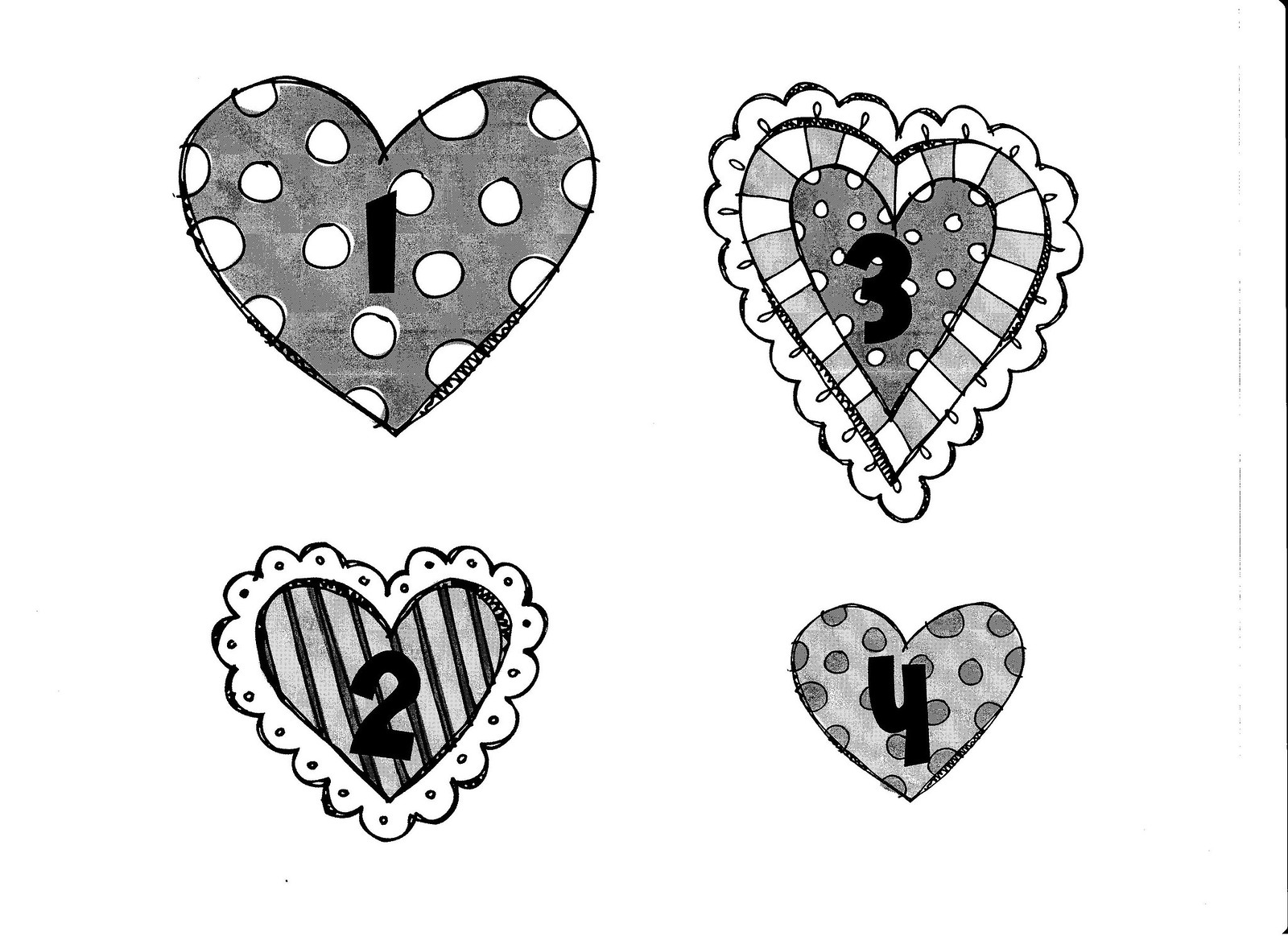This is a detailed black-and-white ink drawing of four distinctly patterned Valentine's hearts, each labeled with a bold number. The top-left heart, labeled "1", is large with a gray background adorned with white polka dots. Below it, the heart labeled "2" features a light gray interior with dark diagonal stripes and is surrounded by a white, lacy, frilly border. To the top right, the heart labeled "3" is dark gray with white polka dots, outlined first by alternating light and dark stripes, and then by a frilly border. Finally, the bottom-right heart, labeled "4", is light gray with dark polka dots. The image emphasizes the contrasting patterns and textures within each heart, all drawn meticulously on a plain white background.